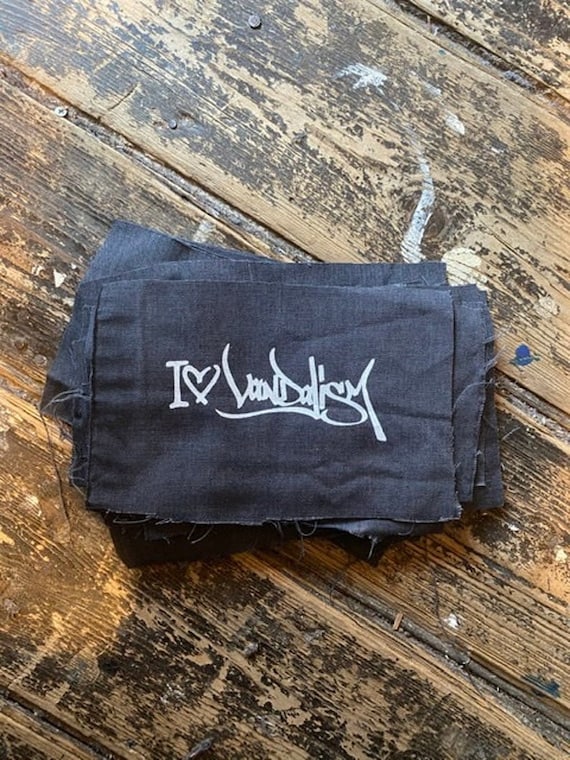The image showcases a detailed, textured scene featuring a pile of roughly cut, rectangular fabric pieces that appear to be either dark denim or a light black material. These fabric swatches, approximately 10 to 20 in number, are stacked haphazardly on an old, worn wooden surface. The wooden background, possibly a table or floor, is notably distressed, with visible paint splotches in white, yellow, and blue, and large sections of the original brown paint worn away to reveal the bare wood beneath. The top piece of fabric prominently displays the text "I ❤️ Vandalism" written in white. The overall color palette of the image is neutral, dominated by shades of black, white, and brown. Additionally, the fabric pieces have frayed edges with threads sticking out, adding to the scene's rustic and neglected aesthetic.